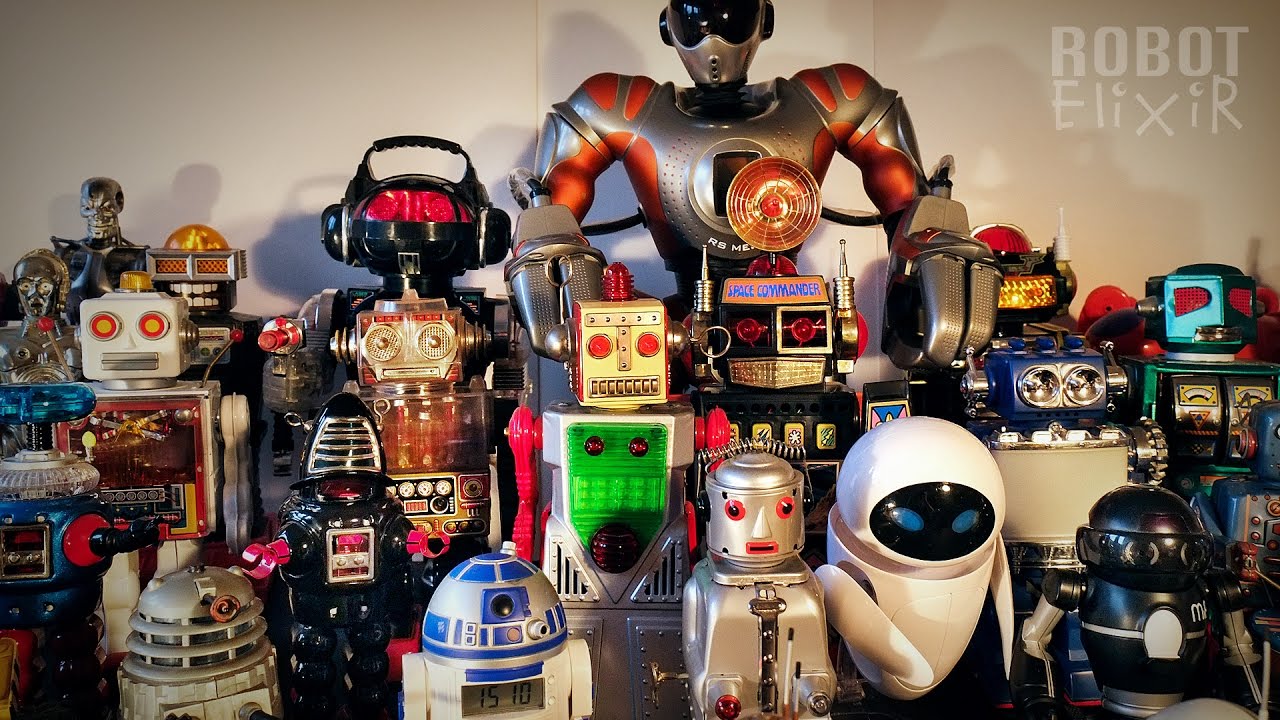In this image taken in warm, low lighting, dozens of colorful robot toys are grouped predominantly in the bottom four-fifths of the frame, extending almost to the top. They sit on the floor against a white wall, with "Robot Elixir" written in light gray, uppercase letters in the upper right corner. The eclectic collection includes both vintage 80s styles and recognizable pop culture icons such as R2-D2—displaying "1510" on his screen—C-3PO, and Eve from WALL-E. Noteworthy robots include a blue one with a water spigot-like wheel on its head, a square white-headed robot with red, yellow, and button details, and an expressive black robot with sunglasses and an orange cap. There’s also a tall, silver robot with orange accents and bug-like eyes, and another resembling a ghost with a white body and blue eyes. From a mini black robot with a round head to a "Space Commando" with a propane heater-like top, the diverse array shows an imaginative and detailed array of robots spanning various eras and styles.